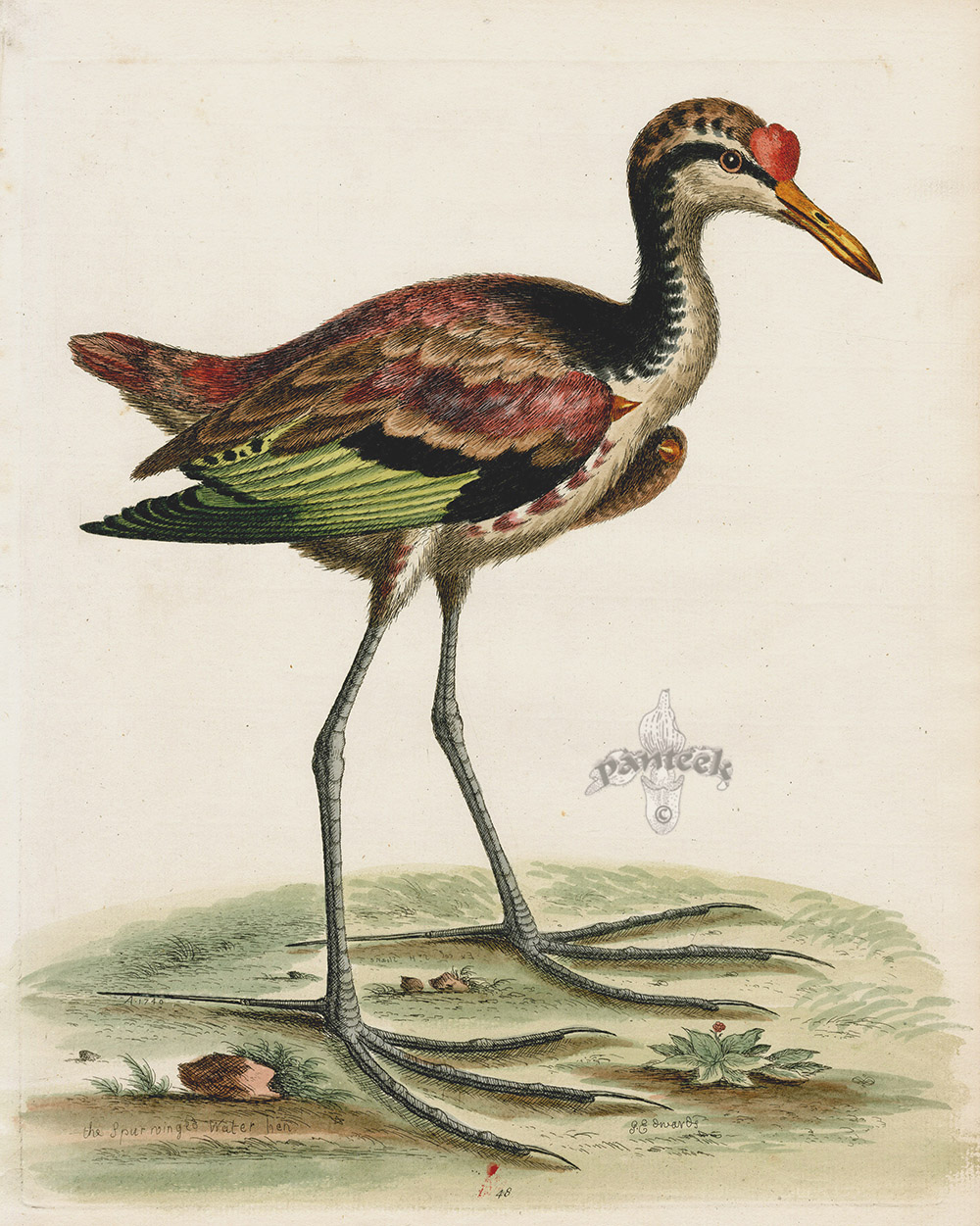Against a light whitish-gray background, this detailed painting of a bird features a striking blend of vibrant colors and intricate details. The bird, reminiscent of an Audubon illustration, stands on a green patch of land and showcases very long, grayish legs with four elongated toes ending in white, sharp toenails, along with a long, sharp projection at the back for balance. The body of the bird is robust, similar to that of a turkey, with a slightly elongated and narrower neck.

The bird is depicted looking to the right, displaying a long, sharp, orange-yellow beak with a small red crest just above it. Its head features an intriguing pattern with orange and black spots and a distinct black line running from the beak through the eye area, merging into a larger black area at the back of the neck. The front and chest area are colored in grayish-white.

The wings exhibit a layered pattern of brown feathers with some red highlights, while the lower tail feathers are a mix of olive green. Additional details include a name, "Pantic," set against the light lavender background, suggesting the artist's signature. The overall use of colored pencils lends a textured, rich quality to the painting, highlighting the skill and effort put into creating this lifelike representation of the bird.